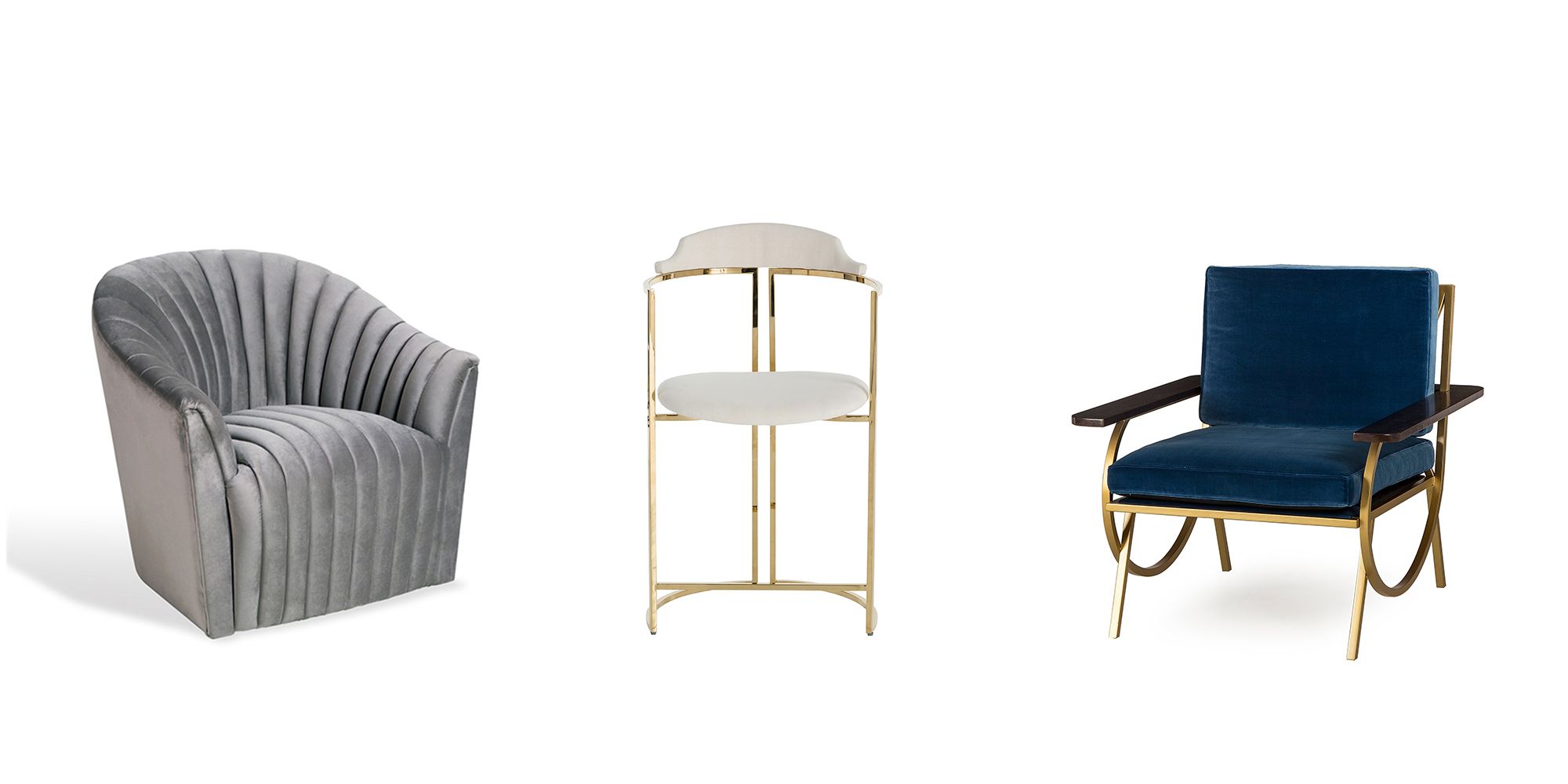This is a photographic image featuring three distinct pieces of furniture set against a plain white background. On the left is an upholstered easy chair, finished in a grey ribbed fabric with armrests and a wingback design, positioned diagonally from the top left to the bottom right corner, exuding comfort and an inviting appearance. In the center, there is a decorative stand with three metal legs, gold in color, supporting two trays, one on the lower shelf and another on the upper shelf, suitable for displaying curios or statues. On the right is a chair with a more structured, almost office-like design, featuring four metal legs, golden brown armrests and legs, with an off-white or cream-colored stiffer upholstery, and a blue cushion for added comfort. The scene lacks any text, keeping the focus solely on the furniture pieces.